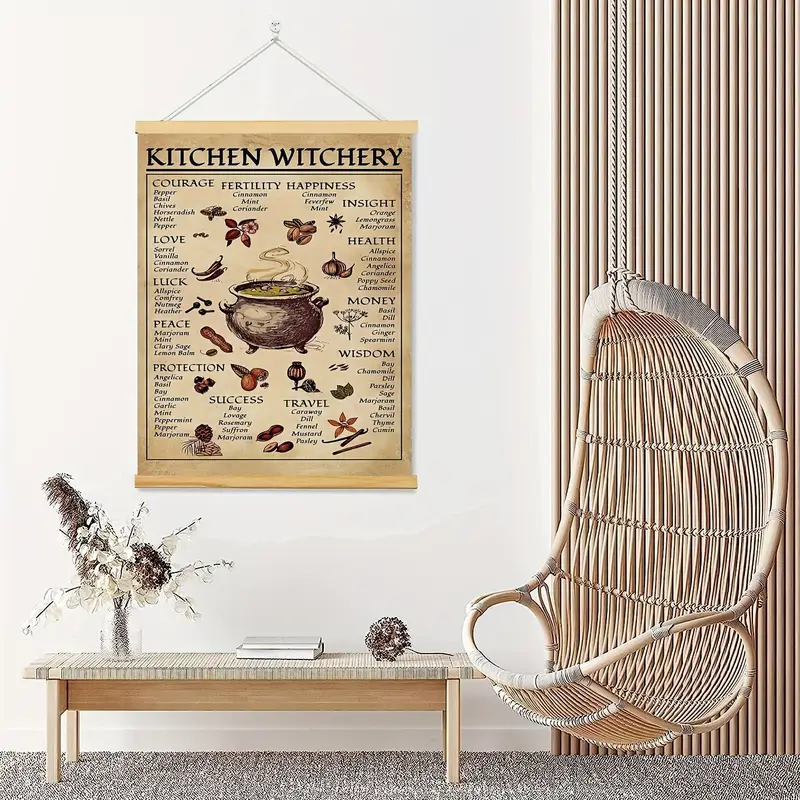In this cozy indoor room, a suspended wicker chair hangs gracefully from the ceiling by sturdy white ropes, adding a touch of rustic charm. The chair, woven from light-colored wood, floats above a soft, gray carpet that grounds the space. To the right of the chair, a white wall showcases an intriguing, scroll-like tapestry pinned up by a string. This aged paper banner, titled "Kitchen Witchery," features a central cauldron with a boiling green potion and a cloud of vapor, giving it a mystical feel. Surrounding the cauldron are words like "Courage," "Fertility," "Health," "Money," "Wisdom," "Travel," "Success," "Protection," "Peace," "Love," "Luck," and "Insight," alongside drawings of various ingredients such as nuts, green leaves, garlic, and peppers, presumably associated with these virtues.

Beneath the tapestry, a small wooden bench stands against the wall, serving as a functional yet decorative element. This light wooden bench holds a clear vase filled with white flowers, flanked by a stack of two books and a mix of brown and white dried plants, adding a touch of natural beauty. The minimalistic design of the bench and its contents complement the serene atmosphere of the room. Adjacent to this display, the wall features long, thin wooden strips lined up side by side, echoing the natural materials and earthy tones seen throughout the space. The room's serene, witchy ambiance is elegantly captured in this scene, blending functionality with a touch of enchantment.